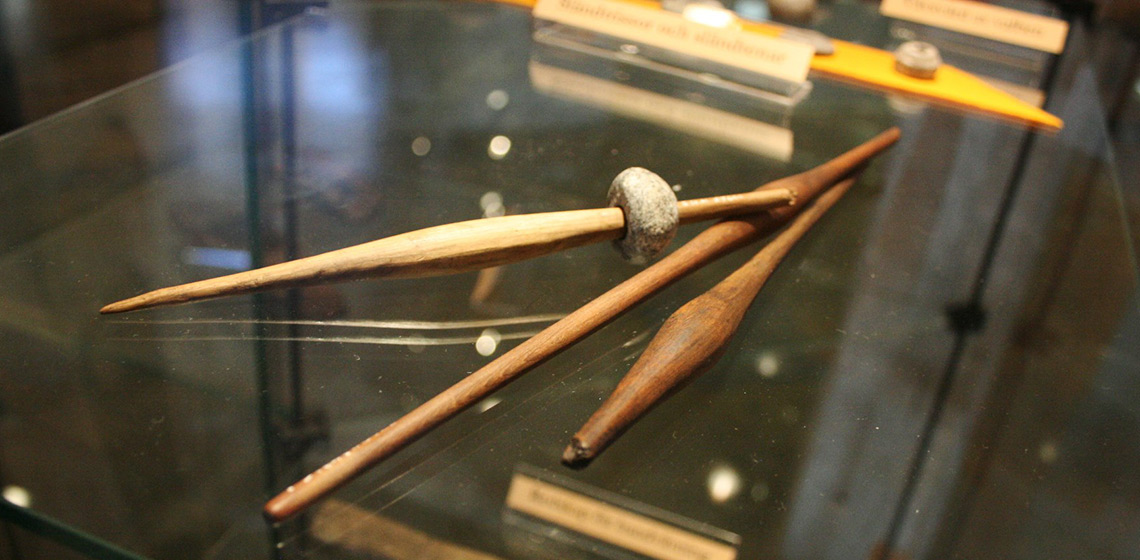This photograph depicts a display case featuring three vintage wooden spindles, tools historically used in the textile industry for spinning fibers into thread. The spindles, crafted from wood and showing various stains, exhibit unique characteristics: each tapers at both ends and is wider in the center, with intricate carvings and a time-worn patina. Positioned on a reflective glass surface, catching the light, these spindles also feature a circular area essential for drawing and twisting fibers into thread. One spindle intriguingly has a piece of rock or clay wrapped around its end, adding to the collection's rustic charm and historical intrigue. The display is set against a backdrop featuring additional wooden elements, possibly part of the setup, enhancing the vintage aesthetic and providing context for these fascinating tools of the past.